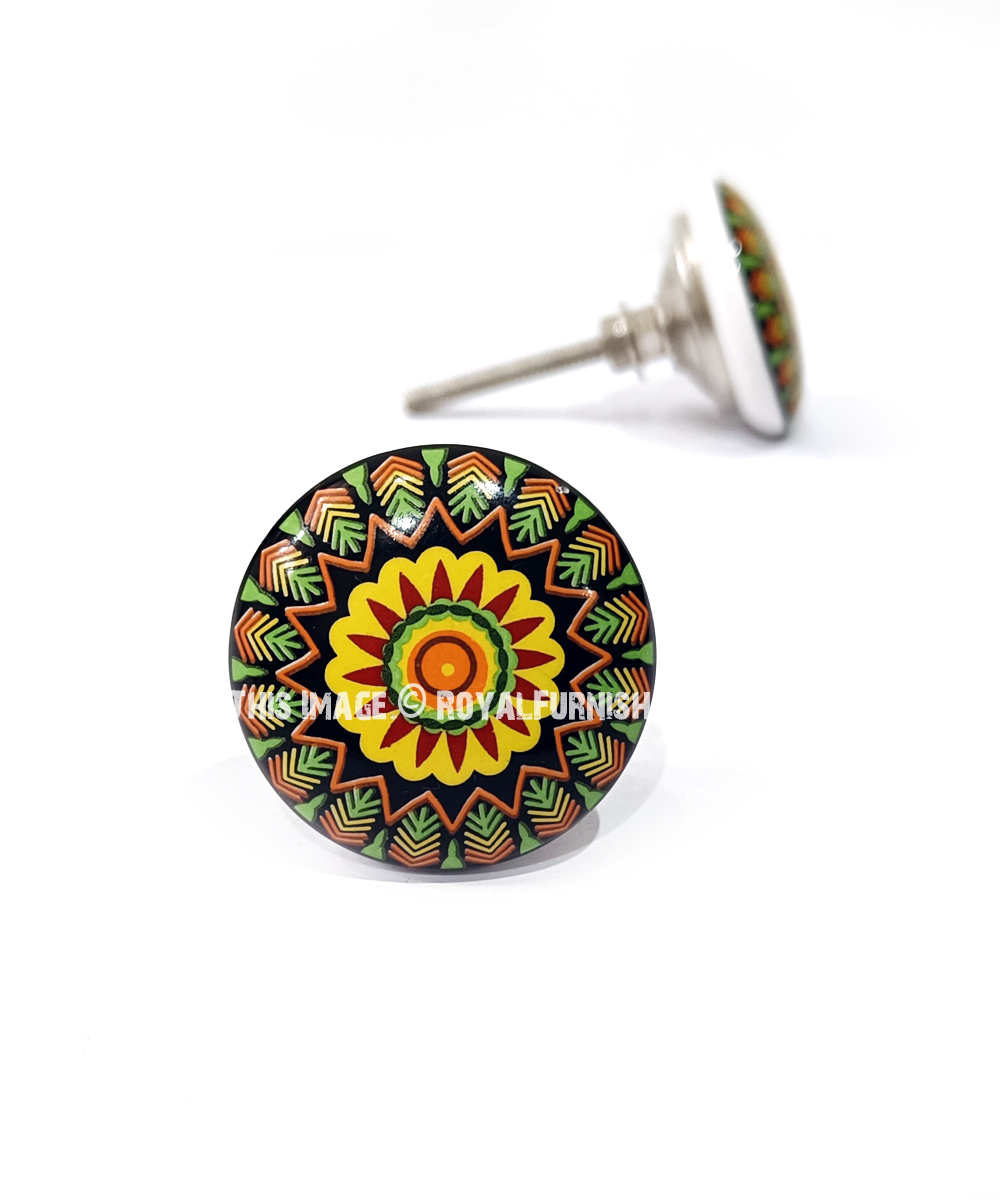This image features two post earrings showcased with the text "HS" or "HIS image at Royal Furnish" overlaid. The earrings exhibit an intricate, colorful, and kaleidoscopic design. Each earring has a ceramic top with a black background, displaying a detailed and vibrant pattern. At the center, a yellow dot is surrounded by a maroon circle and an additional larger orange circle. This is further adorned with geometric designs including yellow blossom-like shapes with burgundy triangular petals, green and yellow circles, and a star-shaped orange array with approximately 15 to 20 points. Between these points are fern-like shapes in green, yellow, and orange. The first earring is positioned in the background, slightly blurry, while the second earring is more prominent in the foreground. The overall aesthetic highlights a rich mix of blacks, oranges, yellows, reds, greens, grays, and whites, creating an eye-catching display.